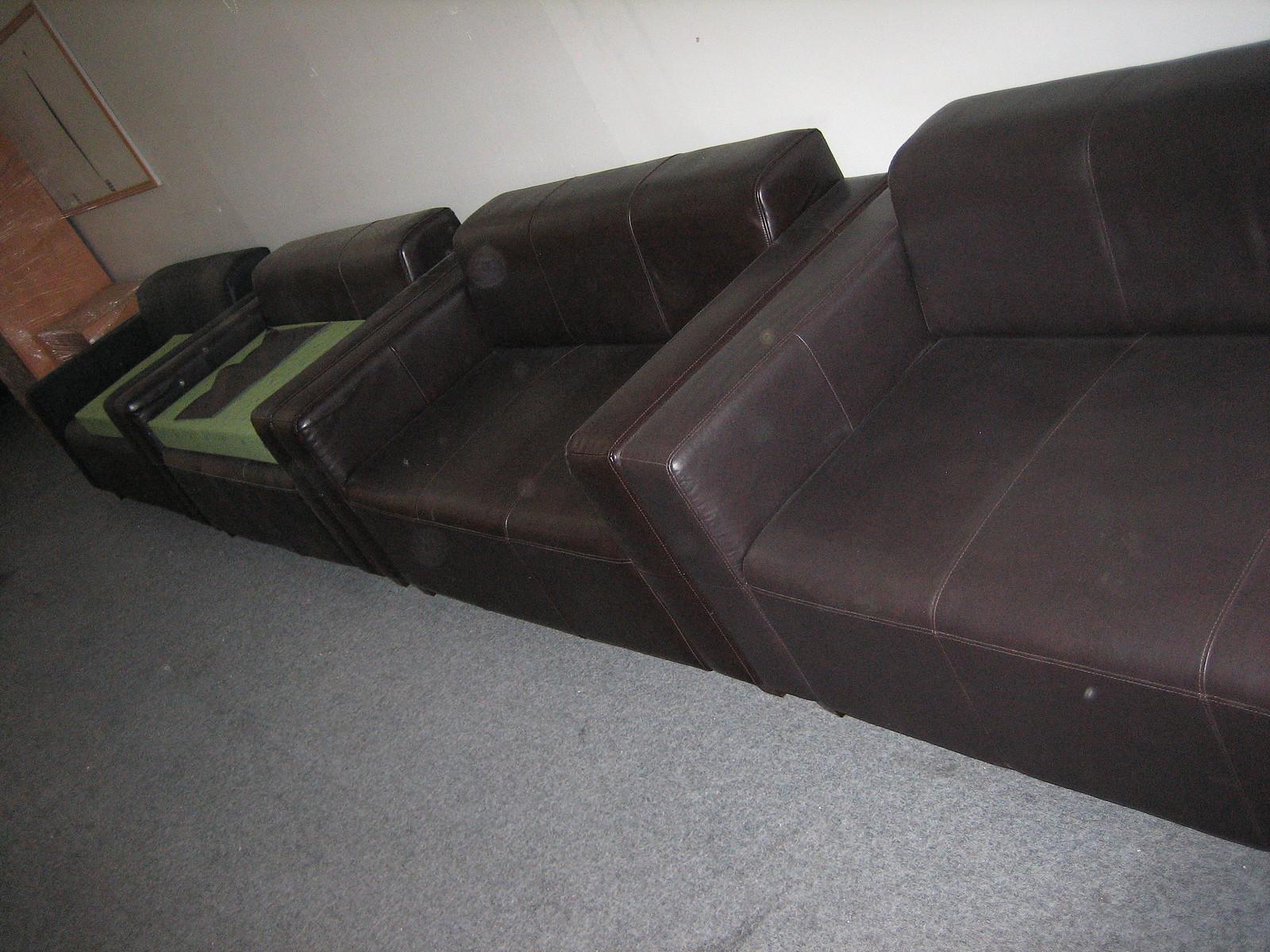The image depicts a room with a row of four identical dark brown leather loveseats positioned against a beat-up white wall. They sit on gray speckled concrete flooring, which resembles indoor-outdoor style carpet. The loveseats feature slightly rounded arms. Two of the loveseats have thick green foam pieces placed on their seats, one of which also has a dark brown piece of fabric resting on it. In the background, there appears to be additional wood furniture wrapped in clear plastic wrap, and a whiteboard with an oak-colored frame is mounted on the wall near this furniture.